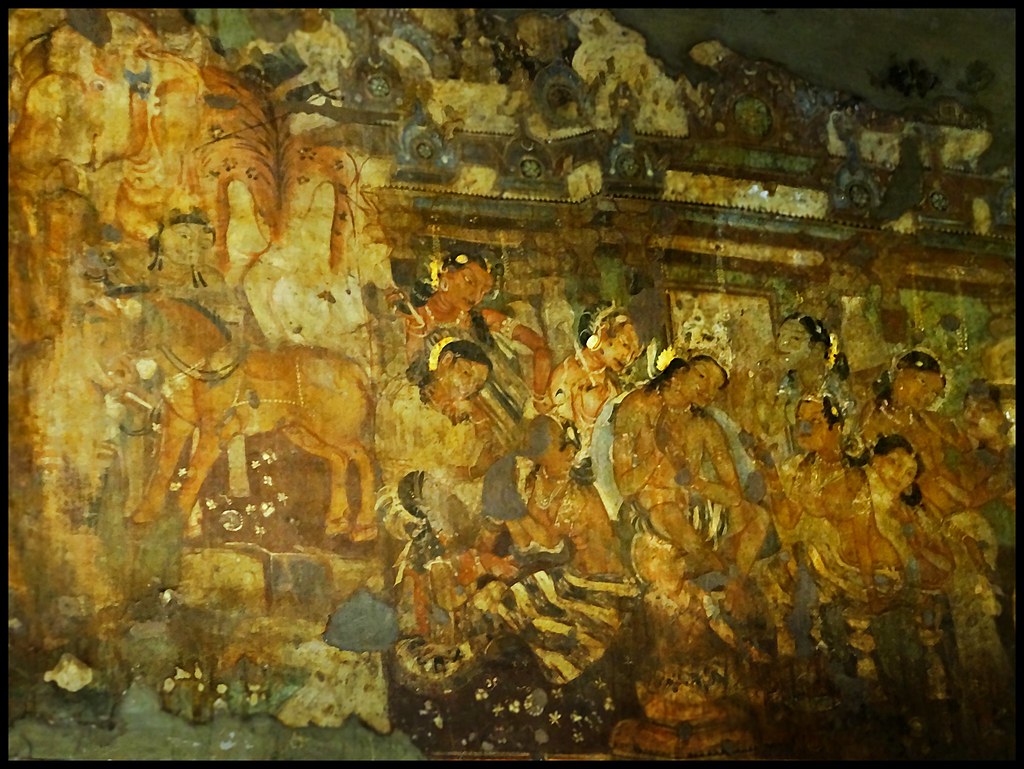This ancient, faded oil painting, likely from India, depicts a religious or royal scene set against an old temple wall. The central figure, possibly a king or religious leader, wears a golden crown and is surrounded by women adorned with crowns, all of whom have dark skin and black hair. These women, some heavily garbed in black and gold skirts, seem to be attending to the central figure. The painting's hues are dominated by oranges, yellows, and dark browns, and the figures themselves appear orange. The scene includes a building with a green roof and windows in the center and right part of the painting. On the left-hand side, a small brown pony faces left, and there are other indistinct animals that might be lions or other creatures. The painting shows signs of significant age, with parts of it faded and chipped away.